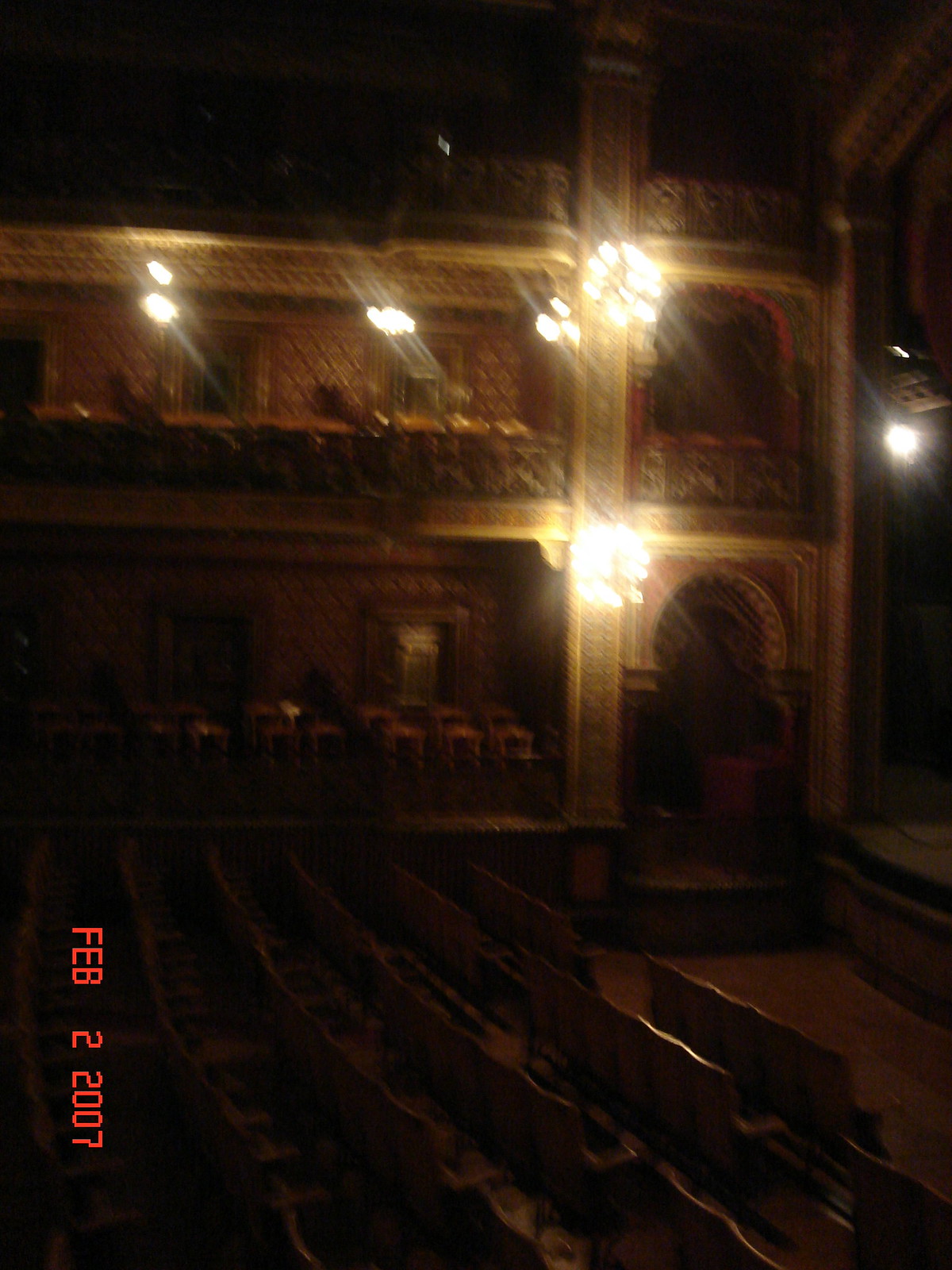This haunting photograph captures the interior of an old, regal Broadway theater late at night, moments before closing. The image is slightly blurry and bathed in darkness, intensifying its eerie atmosphere. Only a few dim lights cast shadows across the ornate, two-story interior, revealing elaborately designed walls, old-time lighting fixtures, and rows of seats with gold-fringed details. The lower portion of the picture faintly shows a stage just to the right and several seats arranged at the bottom. On the far left, a vertical red date stamp reads "Feb 2, 2007," grounding the image in time. Despite the obscured details, the theater's majestic yet creepy ambiance is palpable.